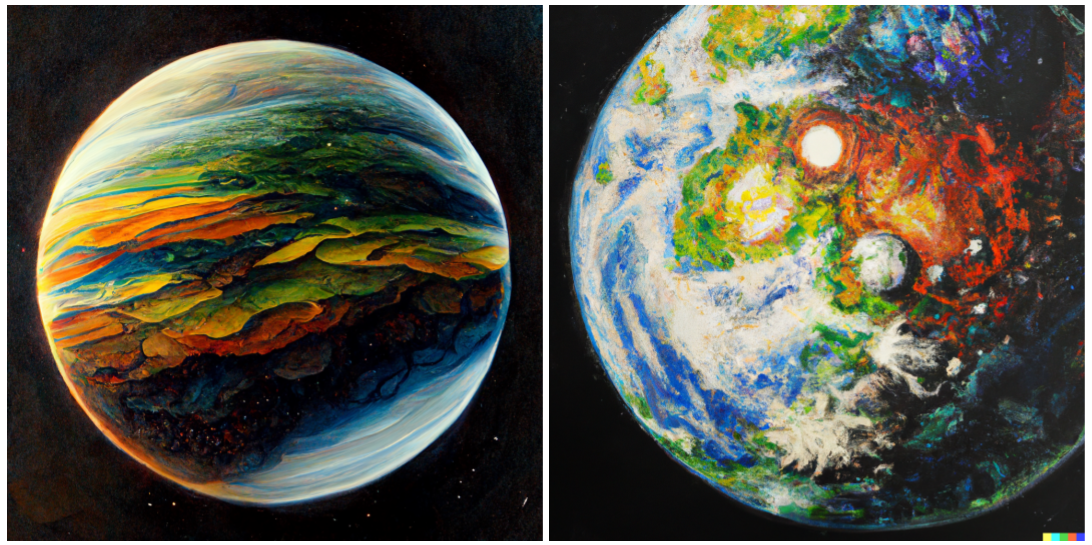The image features two distinct and colorful planets set against a black, star-speckled background, each planet depicted within its respective black-bordered square. 

On the left side, the planet appears richly patterned with horizontal layers in an array of vivid colors. The top part shows a mix of blue shades resembling clouds or water, while the middle section transitions through bands of yellow, orange, and green, interspersed with black rock-like formations. The bottom segment of this planet is a lighter blue, giving it a marbled appearance with swirls intermingling from left to right.

The planet on the right, slightly larger, evokes a celestial body similar to Earth. It features swirling patterns and diverse shapes, contrasting with the smoother lines of the left planet. Towards the left part of this planet, blue and white hues dominate, reminiscent of Earth's oceans and clouds. The right side reveals more dramatic features, including areas of red suggesting volcano-like lava flows, a small white circle, patches of green, and darker black regions. Bright stars can be seen in the bottom left of the image, adding a touch of celestial detail to the scene.